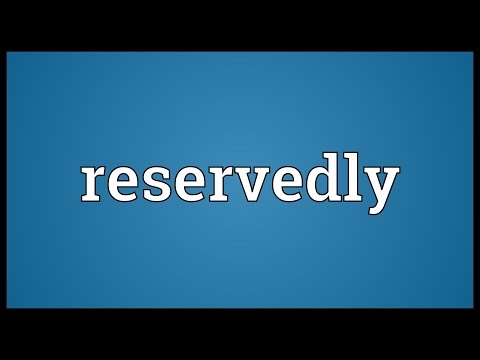The image is a simple, horizontally rectangular depiction with a predominant light to medium blue background. Centered in the middle of this blue rectangle is the word "reservedly" in lowercase white letters, spelled R-E-S-E-R-V-E-D-L-Y. The word is distinctly placed in a typical computer screen font. The blue area extends nearly to the edges on the left and right, leaving only a thin black border on both sides. At the top and bottom of the image, there are thicker black borders, each about 6 to 7 centimeters wide, contrasting against the blue background, which spans most of the image. The overall appearance is neat and solid, with clear, pixelated text that emphasizes the simplicity and clarity of the design.